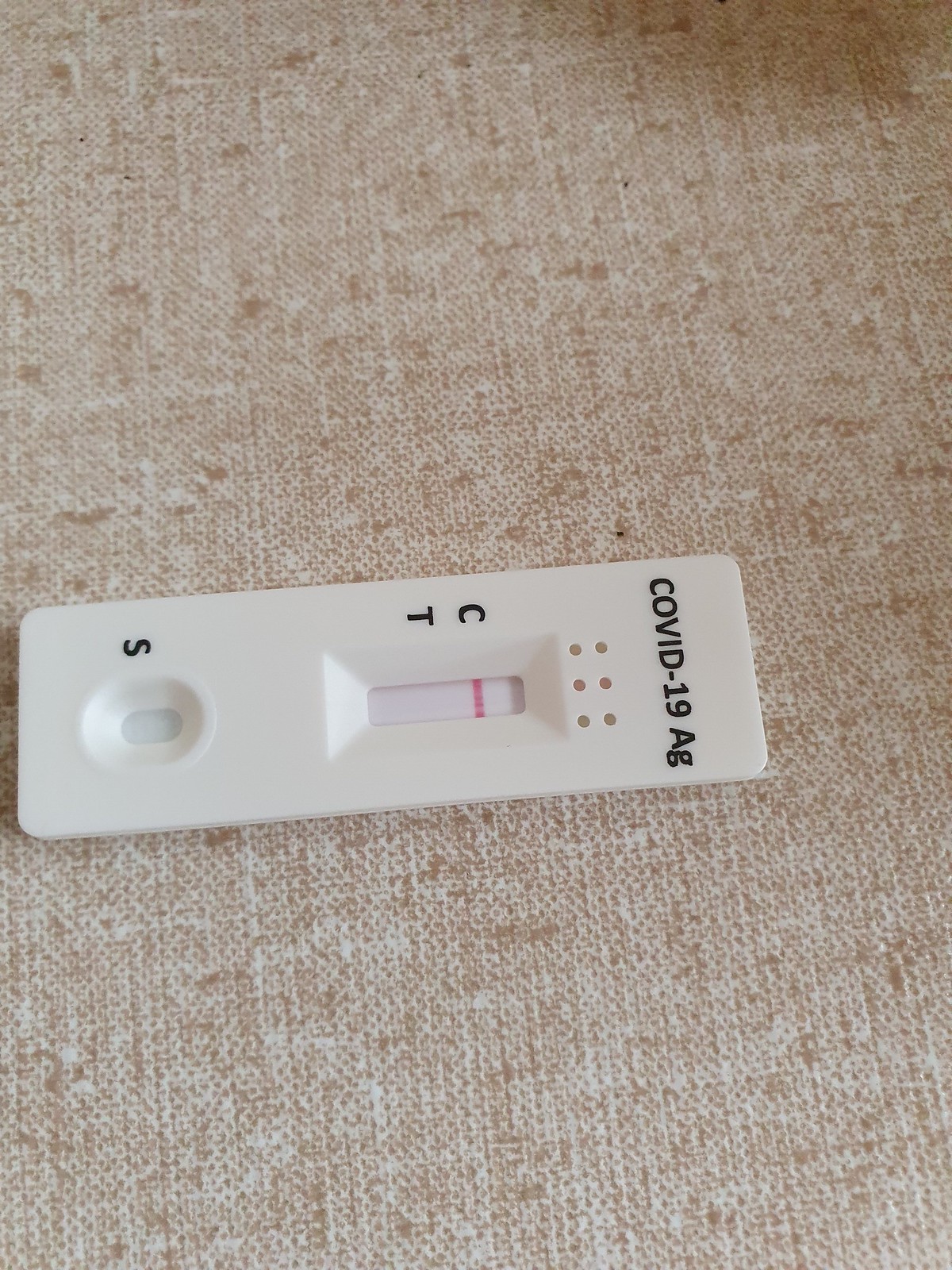This photograph features a COVID-19 antigen test laid out on a light brown and white or taupe fabric, possibly a linen or canvas tablecloth, giving the impression of a vintage table style from the 70s. The white test device prominently displays "COVID-19 AG" at the top and features six small pinprick holes, with the two central holes exhibiting a pinkish hue. At the bottom of the test, there is an oval-shaped well with a bluish tint for placing the fluid drops, marked with an "S" nearby. The test result area features markings "C" (control) and "T" (test). In this image, only the "C" has a pink line, indicating a negative result for COVID-19.